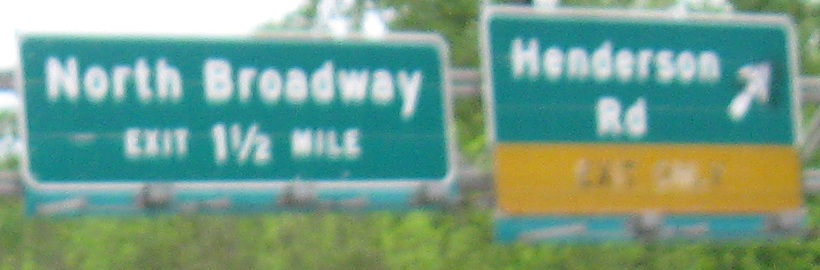This photograph captures a pair of green highway road signs against a backdrop of light green foliage from distant trees and a cloud-covered, white sky. On the left, the rectangular sign reads "North Broadway, Exit 1 1/2 Miles" in white print, held up by metal poles. To the right, there's a taller, more square-shaped sign that reads "Henderson Rd" with a white arrow pointing diagonally to the upper right, indicating an exit. Underneath the Henderson Road sign, a yellow-bordered banner states "Exit Only." Though the image quality is blurry, the details of the signs and the overcast day's effect on the sky and surrounding trees are still discernible.